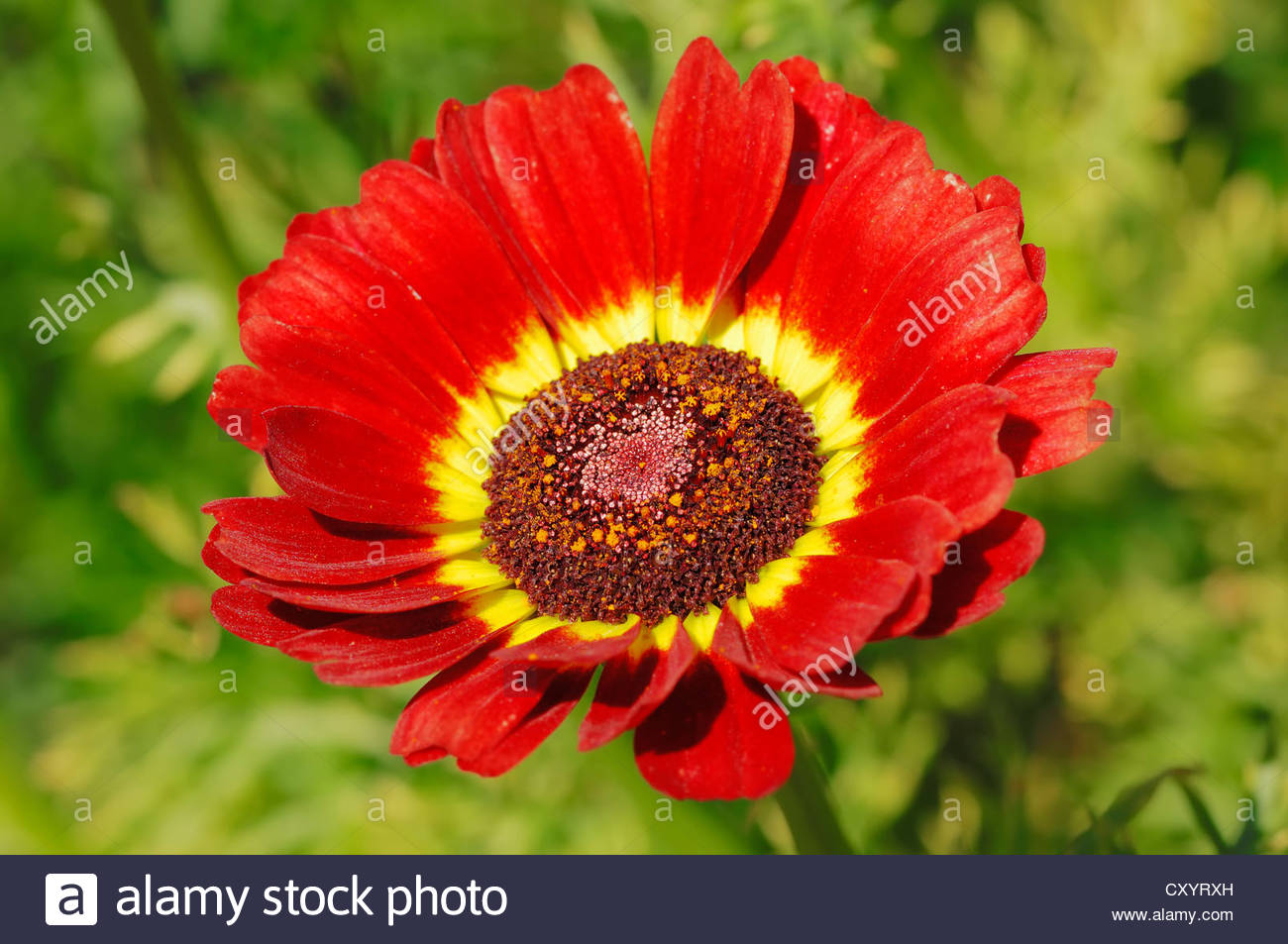The image is a close-up, horizontal rectangular photo of a fully bloomed red flower, which is centrally placed within the frame. The flower features multiple narrow, tall, red petals, each with a yellow base that appears like a small yellow flame, forming a prominent yellow ring around the brown-amber pollen area in the center. The perspective of the shot is slightly angled, with the lower petals appearing at the top of the image and the uppermost petals at the bottom, revealing a bit of the flower's interior. The background consists of blurred green vegetation, enhancing the flower's vivid colors but rendering the surrounding foliage indistinguishable. The green stem of the flower is visible in the bottom center of the image. A noticeable black strip runs along the bottom edge of the photo, including a logo featuring a lowercase 'a' in a white box, followed by the text "Alamy Stock Photo," and smaller, harder-to-read text that includes a potential URL and possibly "C-X-Y-R-X-H." Watermarks with the word "Alamy" often paired with lowercase 'a's are dispersed diagonally across the image, indicating copyright.